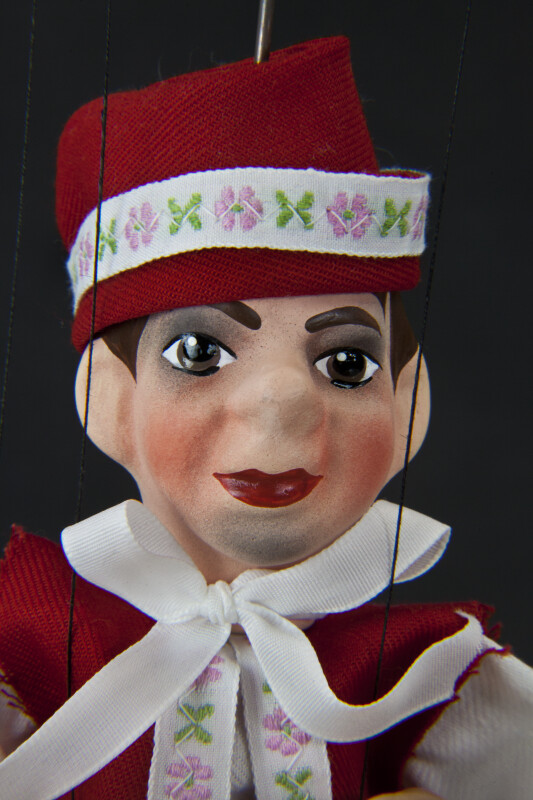This close-up photo features a detailed string marionette with a light Caucasian complexion, set against a black background. The marionette is crafted in the likeness of a man, adorned in traditional European attire. He wears a striking red hat adorned with a floral band—a white border embellished with pink flowers and a green butterfly. His expressive face is accentuated by thick, dark brown eyebrows, big brown eyes with gray eyeshadow, and pink cheeks. His brown hair peeks from beneath the hat. The outfit complements the hat, consisting of a red and white uniform with a prominent wavy white bow under the chin. The red jacket features a sash with a similar floral and butterfly pattern, while the undergarment is white. The marionette is controlled by strings visible on the sides of its face, with a thin metal bar on top of its head.